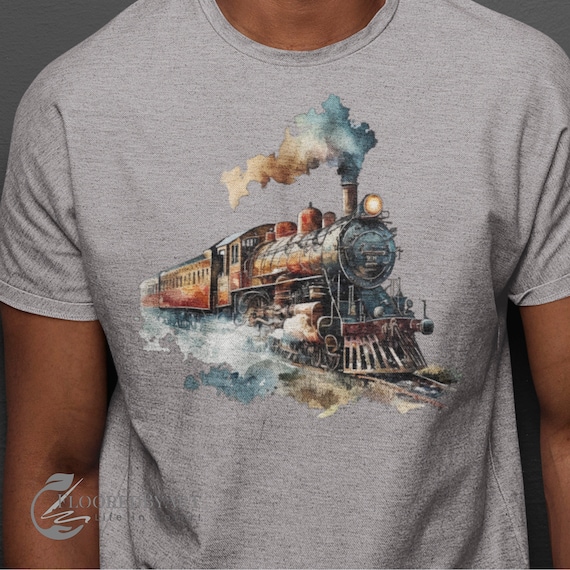In the image, a man with an olive skin tone is wearing a gray short-sleeve U-neck t-shirt adorned with a distinctive graphic. The graphic features an illustrated train rendered in a watercolor style. The train is silvery brown with a prominent red grate at the bottom as it travels over the rails. Blue smoke billows from the funnel at the top, transitioning to gray as it drifts back. Attached to the train is a long reddish-yellow car. In the bottom left corner of the image, a logo with a bluish river and a grayish swoop beside it can be partially seen. The logo appears to say "Florida," although the text is difficult to read as it blends into the color of the shirt.